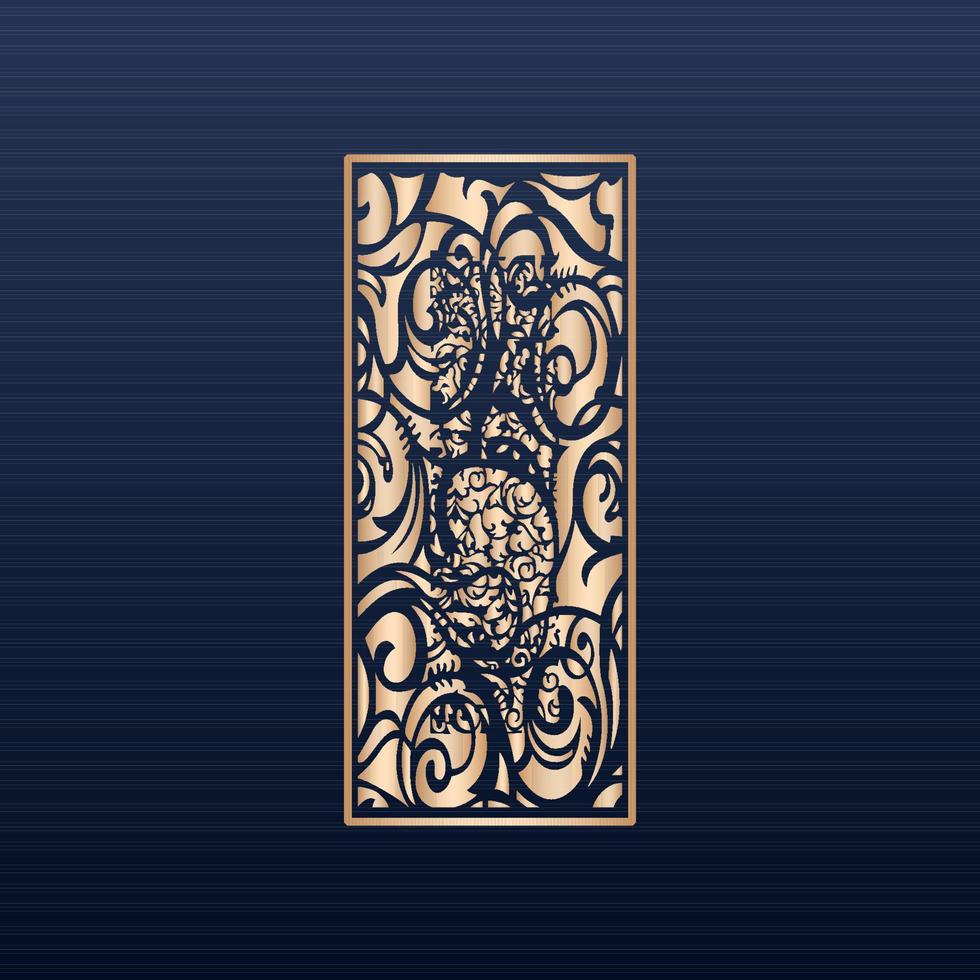The image showcases a striking piece of art set against a dark blue background interspersed with very thin light blue and light gray horizontal stripes. At the center, a decorative element framed by a contrasting white-to-gold rectangle captures attention. This elaborate centerpiece, akin to a filigree design, combines an intricate array of gold puzzle-piece elements that interlock to form an abstract shape resembling a tree. The cutouts within this gold block reveal the dark blue background, intricately forming many small leaves and designs. The combination of delicate lines, contrasting colors, and ornate patterns creates a visually captivating and richly detailed composition.